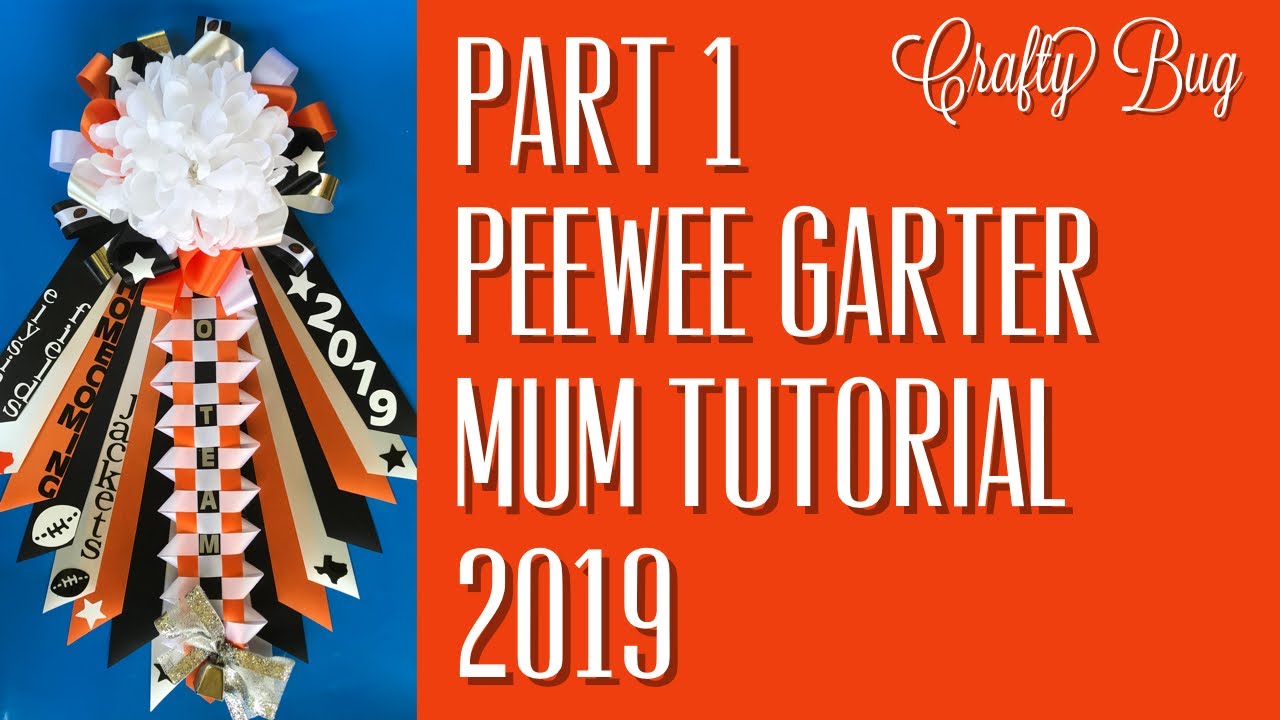This image is a graphic poster from Craftybug, designed with a distinctive two-tone background. The left one-third section is blue, while the right two-thirds section is an orange-red gradient. The orange area features white text that includes "Craftybug," "Part 1: Pee Wee Garter Mum Tutorial 2019." Dominating the blue section on the left, there is a ribbon with a white mum flower at its center. The ribbons cascading from the flower are various colors—black, white, and orange, with intricate designs including one featuring a silhouette of the Texas state map, indicating a connection to Texas. The ribbons bear inscriptions such as "Alyssa Fields," "Homecoming," "Jackets," and "O-Team 2019," and are decorated with a gold bow at the bottom. The detailed and colorful design suggests an advertisement or tutorial poster, possibly for a crafting website.